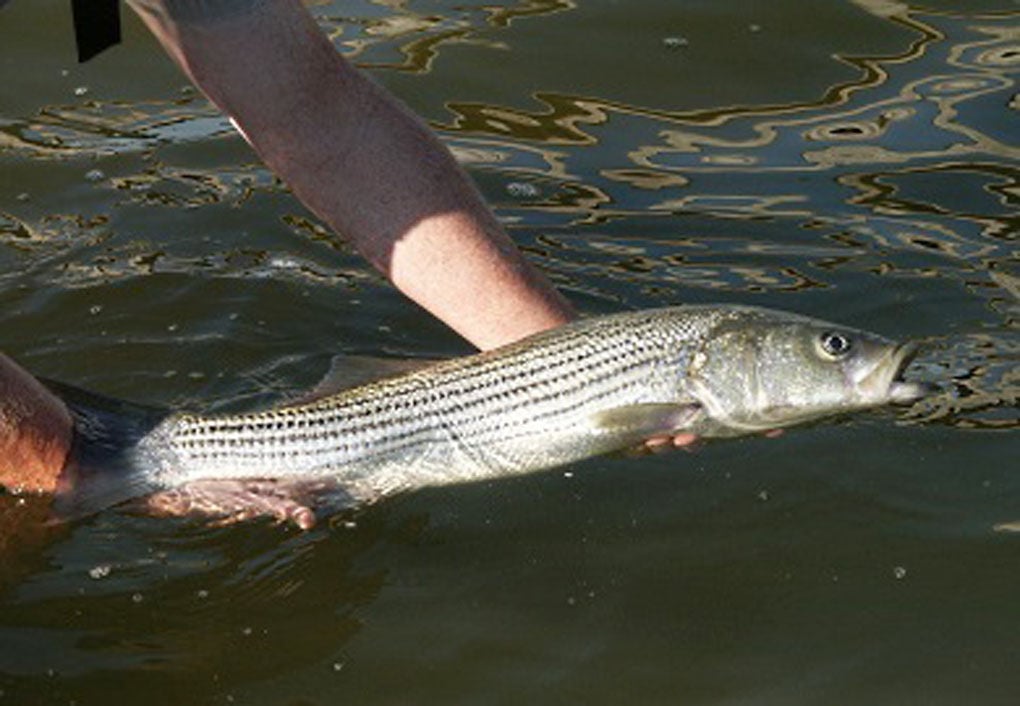In this outdoor color photograph, we see the arms of a man extending from the left side of the frame, holding a long, silver fish just above the murky, brownish-blue river water. The fish, which is almost as long as the man's forearm, is suspended horizontally with its eye and open mouth facing to the right and its tail partially submerged in the water. The fish's body glistens in the light, revealing dark scales along its side and back. The man's arms, caught in the act of lifting the fish out of the water, are the only visible part of him, emphasizing the fish and its shiny, scaly details against the dark, reflective surface of the river.